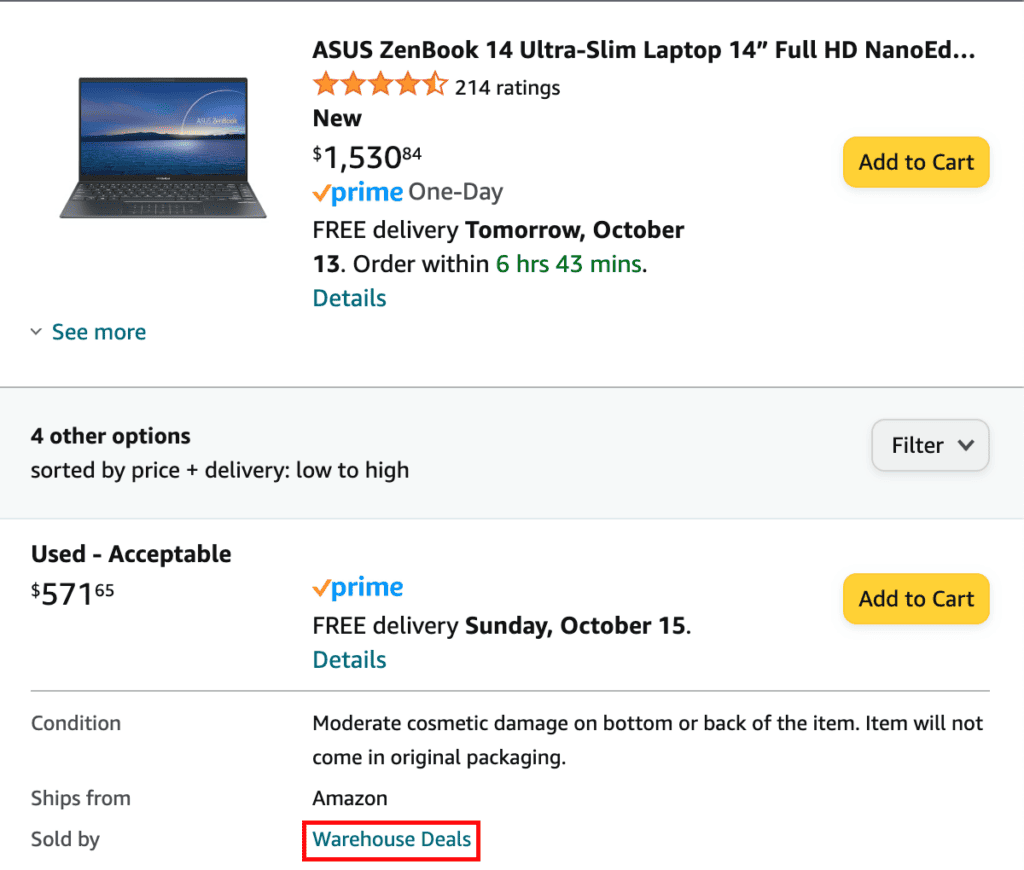This is a cropped screenshot of a product listing from the Amazon website showcasing the Asus ZenBook 14 Ultra Slim Laptop. The laptop features a 14-inch Full HD NanoEdge display. The product title is prominently displayed at the top center of the screenshot. Directly below the title, on the bottom left, there is a 5-star rating indicator accompanied by "214 ratings" to its right.

Underneath the rating, the word "New" is highlighted in bold black letters. Following this, the price is listed as $1,530.84. Beneath the price, it is noted that the product is eligible for "Prime One-Day" delivery, with "Free delivery tomorrow, October 13th" if ordered within 6 hours and 43 minutes. There is a "Details" link at the bottom left for further information.

To the right of this section, a yellow "Add to Cart" button is displayed in black letters. On the left side of the screenshot, there is a thumbnail image of the front of the laptop, with a "See more" link below it.

Toward the bottom of the screenshot, a gray box contains additional options and sorting information. In the top left of the gray box, it says "4 other options," followed by the sorting criteria "Sorted by price + delivery: Low to High." To the right, a drop-down box labeled "Filter" is available.

Below, a secondary listing is shown for a "Used - Acceptable" condition of the laptop priced at $571.65 with "Prime Free Delivery Sunday, October 15th." There is a "Details" link on the bottom left of this section. To the right, another yellow "Add to Cart" button is displayed.

At the bottom of this secondary listing, it says "Condition" on the left, and on the right, it specifies "Moderate cosmetic damage on bottom or back of the item. Item will not come in original packaging." The item is noted to be "Ships from: Amazon" and "Sold by: Warehouse Deals," with "Warehouse Deals" highlighted in a red box around the blue text.